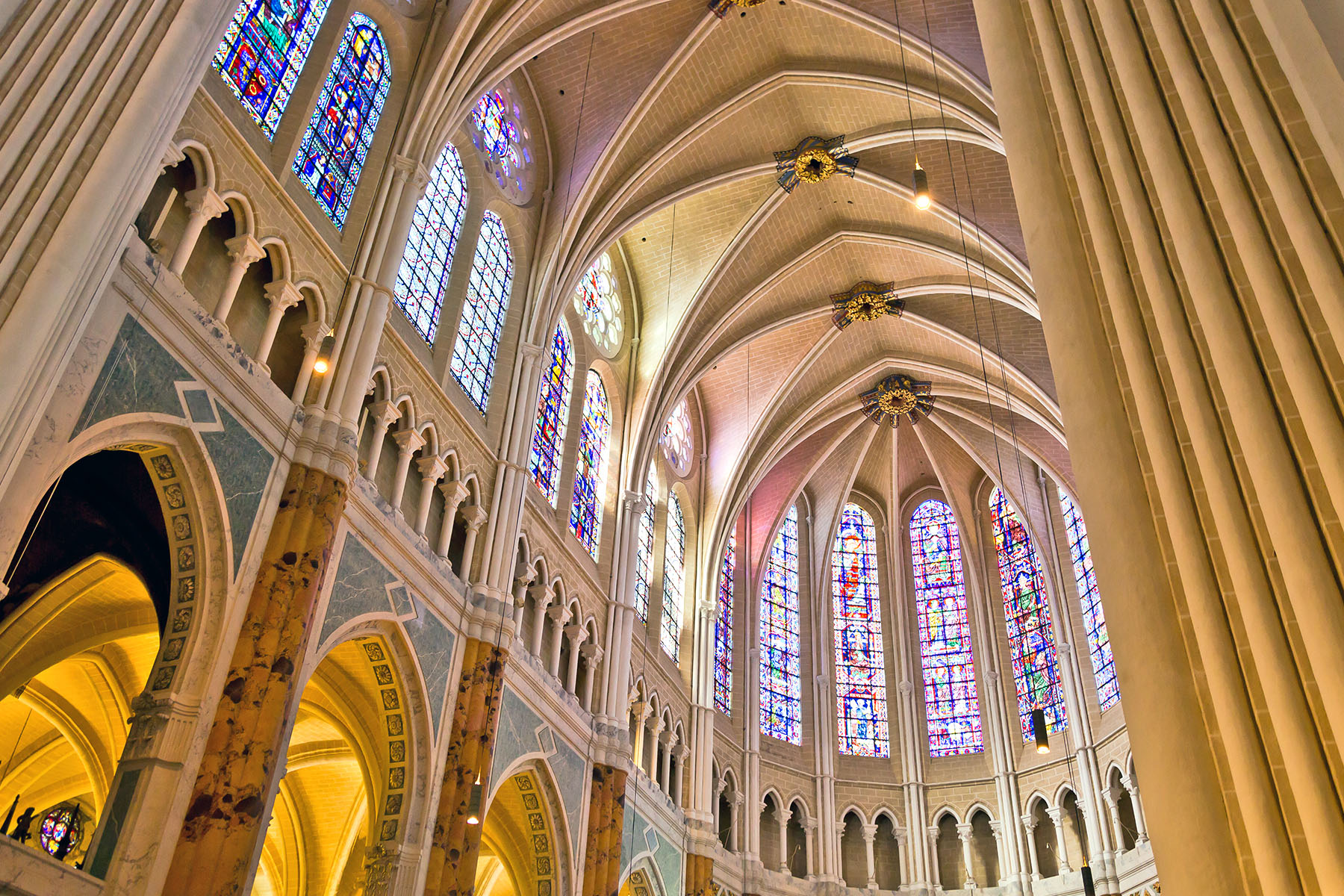This detailed photograph captures the ornate interior of a European cathedral, likely with Catholic influences. The focus is on the ceiling adorned with numerous intersecting arches and support beams, crafted from light stone brick. It's daytime, evidenced by the sunlight streaming through the extensive stained glass windows at the upper part of the ceiling, showcasing vibrant colors including blues, reds, yellows, blacks, oranges, greens, and whites. The top right features marble columns stretching from floor to ceiling, while the left side wall displays a series of arches topped with circular stained glass windows depicting religious imagery. Below the stained glass, the ornate architectural details span horizontally across the image. There's an unexpected addition of a gold curtain or drape falling straight down on the right and a single light bulb hanging from the ceiling. Additionally, one can spot the presence of hallways at the bottom left corner and possibly a few people present, further emphasizing the grandeur and active use of this magnificent cathedral space.